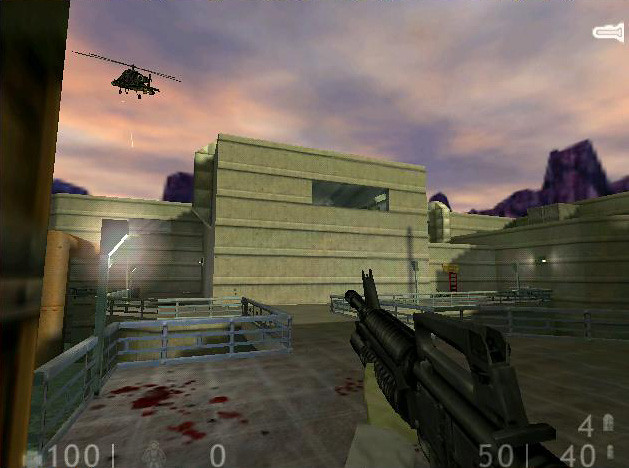This screenshot captures a moment in a first-person shooter video game set in an urban environment characterized by extensive brickwork, metal guardrails, and large concrete buildings. The scene is dominated by a twilight sky painted in purple and pink hues, against which a helicopter hovers in the upper left corner. On the ground to the left, blood splatters hint at recent action. The right side of the screen shows the player's perspective, holding a black assault rifle, with a gloved yellow hand visible. At the bottom of the screen, the in-game stats are displayed: a health or life indicator at 100, a shadowy figure icon at 0, alongside a score of 50, and ammunition counts showing 4 larger bullets and 40 smaller bullets. The image encapsulates the immersive and intense atmosphere typical of modern shooting games.